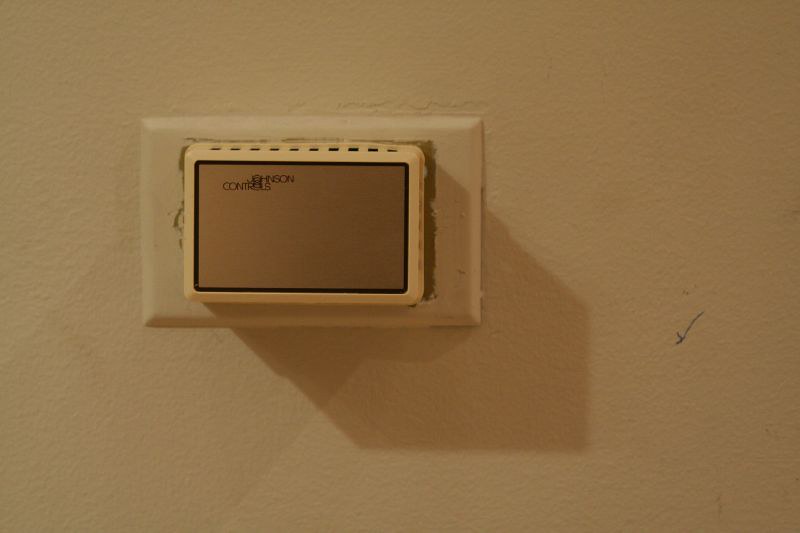This color photograph depicts a rectangular object mounted on another rectangular stand, both seemingly attached to a wall. The image has a yellowish tint, either from artificial lighting or a filter, casting a shadow to the right and bottom of the object, suggesting light from the upper-left corner. The central rectangle features a creamy outline with small black notches at the top, enclosed by a black rim and a brown surface. In the upper-left corner of this area, a black logo is present but unreadable due to its size.

The supporting rectangular stand appears integrated into the wall, protruding slightly, with reflective edges showing. The wall surface has visible textures, and there is a faint scratch or pen mark, suggesting a small arrow pointing diagonally downward towards the center of the image, on the right side of the frame. Besides the prominent shadow from the top-left to bottom-right, a lighter shadow extends in the opposite direction, hinting at an additional light source at the top-right corner.